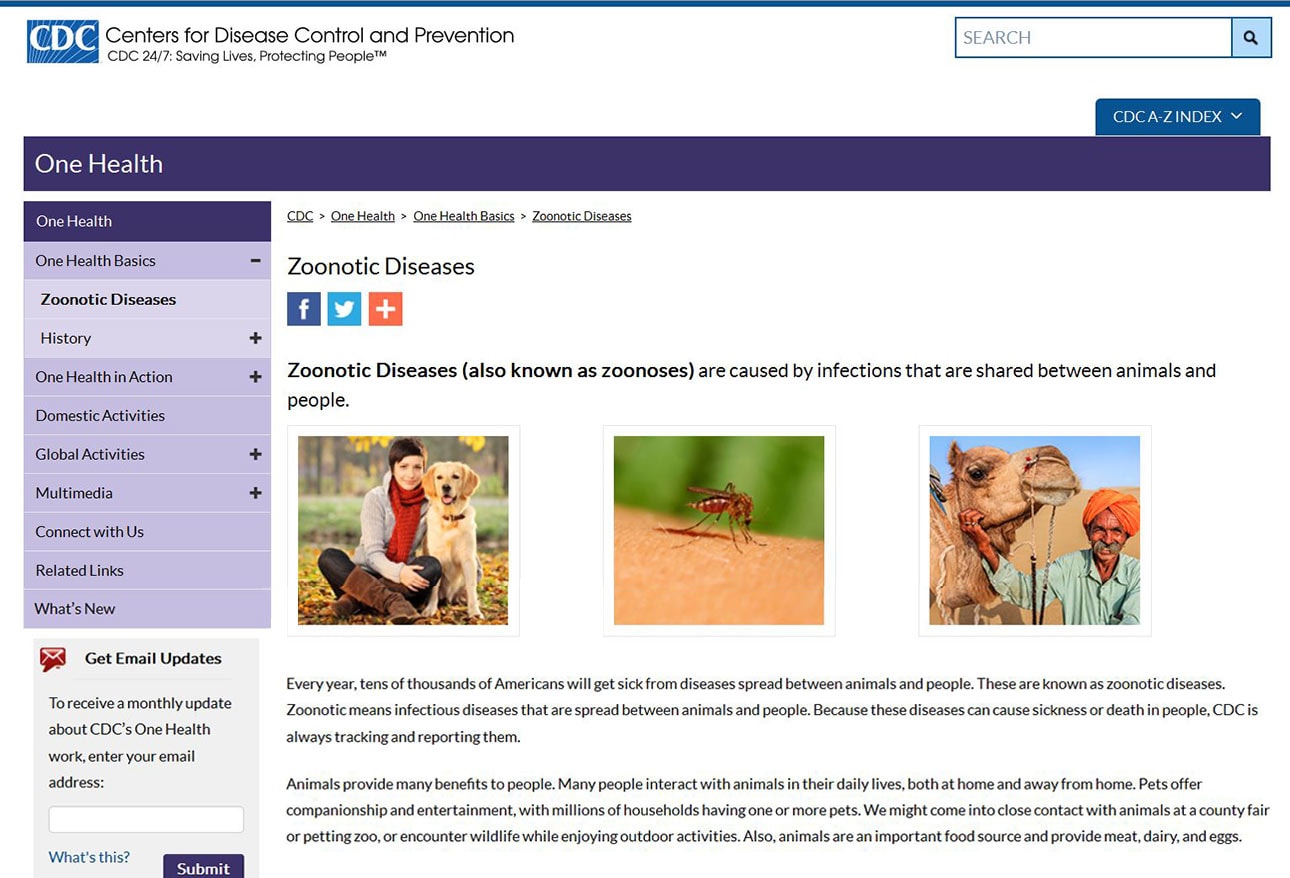A screenshot of the CDC webpage is displayed. At the top, a horizontal gray bar stretches from left to right across the image. Just below this gray bar, on the left side, the CDC logo is prominently featured: it consists of white capital letters in a blue rectangular box, accompanied by the text "Centers for Disease Control and Prevention." Underneath the logo, the phrase "CDC 24/7: Saving Lives, Protecting People" is clearly visible.

To the right of the logo, there is a search engine bar equipped with an input field and a search icon. Beneath the search bar, users can find the "CDC A-Z Index" with a downward-pointing arrow indicating a dropdown menu. Below this, a bold purple rectangle extends across the width of the page, containing the text "One Health" in white.

Directly beneath this header, the website offers numerous categories and options listed vertically: "One Health," "One Health Basics," "Zoonotic Diseases," "History," "One Health in Action," "Domestic Activities," "Global Activities," "Multimedia," "Connect with Us," "Related Links," and "What's New." A section titled "Get Email Updates" follows, containing an input field for email addresses and a prominent red "Submit" button.

On the right side of the page, a vertical menu lists similar categories: "CDC One Health," "One Health Basics," and "Zoonotic Diseases." Below this, social media icons representing Facebook, Twitter, and Google Plus are displayed. Finally, the bulk of the webpage showcases the main content and articles, summarizing the essence of the website.